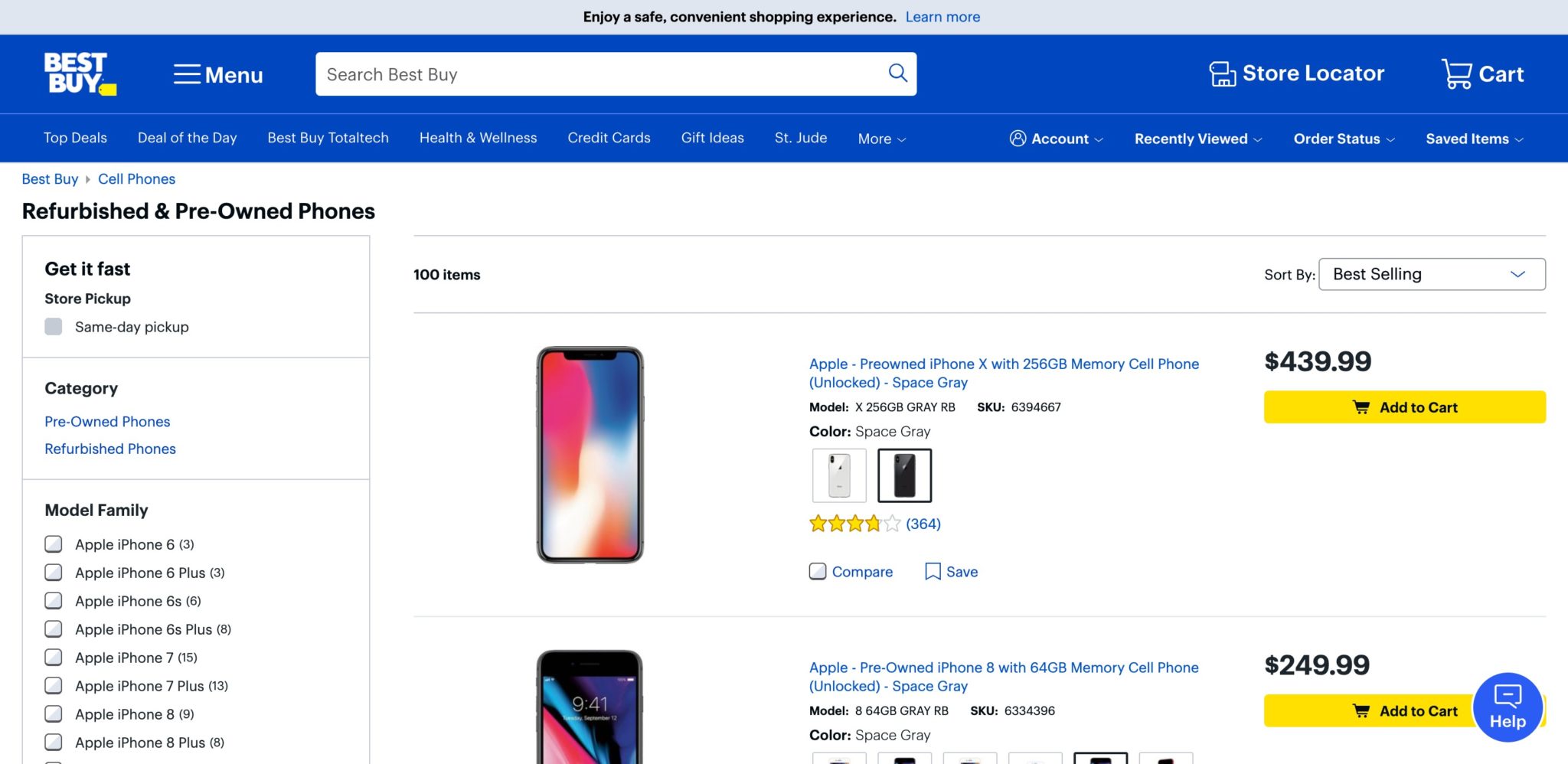The image depicts the Best Buy website interface. At the very top, the recognizable Best Buy logo is displayed inside a yellow price tag icon. Adjacent to the logo is a white search box labeled "search Best Buy" with a blue magnifying glass icon inside it. The navigation bar contains various options including "store locator," "cart," and several tabs such as "Top Deals," "Deal of the Day," "Best Buy Total Tech," "Health and Wellness," "Credit Cards," "Gift Ideas," "St. Jude," and "More." Additional features like "Account Page," "Recently Viewed," "Order Status," and "Saved Items" are also accessible.

The main content of the webpage highlights a section dedicated to "Refurbished and Pre-Owned Phones." Several categories such as "Get it Fast," which includes a checkbox for "Same Day Delivery," as well as "Pre-Owned Phones" and "Refurbished Phones" are listed.

Prominently featured on the page is a listing for an "Apple Pre-Owned iPhone X" with 256GB of memory. The phone is noted as "unlocked" and available in "Space Gray" for $439.39, accompanied by a yellow "Add to Cart" button. Below it, another listing showcases an "Apple Pre-Owned iPhone 8" with 64GB of memory, also "unlocked" and in "Space Gray" for $249.99, and it too includes a yellow "Add to Cart" button. A blue "Help" button is also present on the webpage for customer assistance.